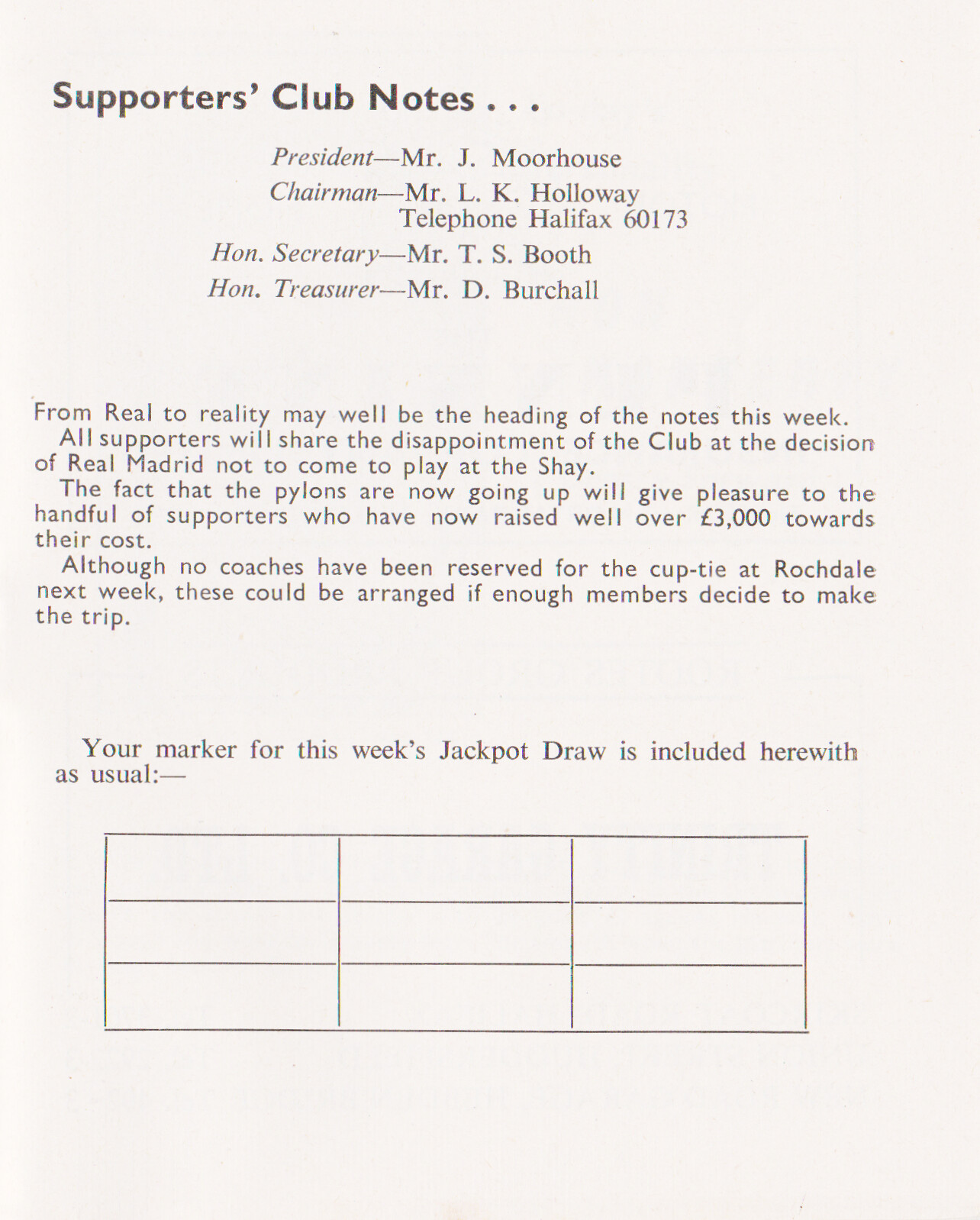The image features an old, tan sheet of paper that takes up the entirety of the frame, set against a white, empty background. The document is titled "Supporters Club Notes" at the top and is adorned with black text detailing various club positions: President Dr. J. Morehouse, Chairman Mr. L.K. Holloway, Honorary Secretary Mr. T.S. Booth, and Honorary Treasurer Mr. D. Birchall, with a contact telephone number listed as Halifax 60173. The main body of the text, possibly titled "From Reel to Reality," expresses the club's collective disappointment over Real Madrid's decision not to play at the Shea stadium. Despite this setback, there is a note of optimism as supporters have successfully raised over £3,000 towards the cost of new pylons being erected. Additionally, the document mentions the potential organization of coaches for a Cup Tie at Rochdale next week if enough members are interested. At the bottom, there is a small table with spaces to fill in text, possibly for additional notes or a draw. The overall look is that of a vintage handout or form intended for club members.